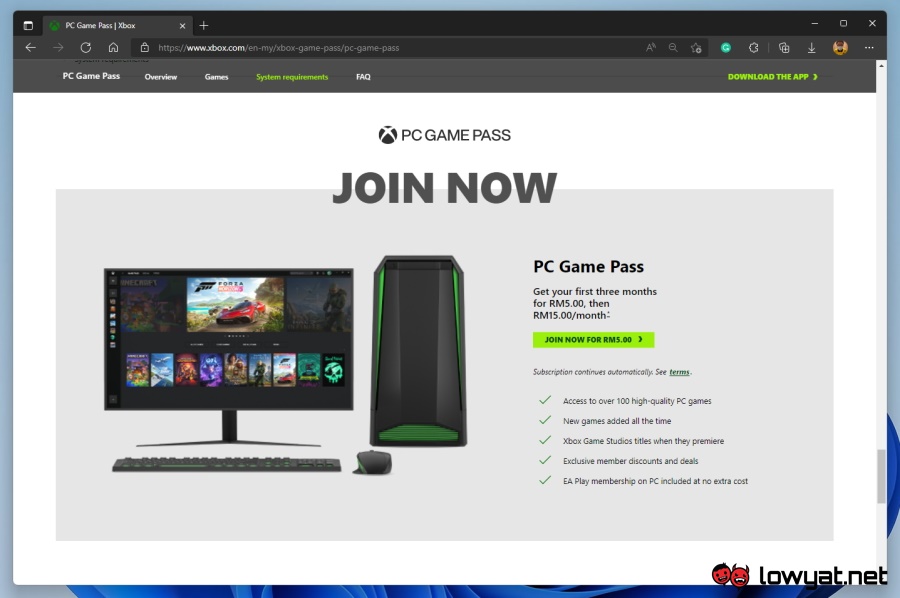This screenshot captures a detailed section of the official Xbox website displayed on a computer monitor. At the top of the page, the browser tab reads "PC Game Pass" while the address bar shows the URL "www.xbox.com", specifically navigating to the subsection for Xbox Game Pass dedicated to PC gaming.

The website's interface is organized with several tabs, including "Overview", "Games", "System Requirements", and "FAQ". The "System Requirements" tab is highlighted in green, indicating it has been selected, with the other tabs remaining in blue. To the far right of these tabs, there is an option labeled "Download the App," accompanied by a right-pointing arrow icon.

Below the navigational menus, a prominent image of a desktop computer setup is featured on the left side of the screen. The setup includes a monitor mounted on a pedestal stand, a keyboard, and a mouse. Positioned beside the monitor is a computer tower. The page also showcases a banner that prominently displays the text "PC Game Pass" along with a call-to-action button inviting users to "Join Now" for RM5 or $5, suggesting an introductory offer for the service.